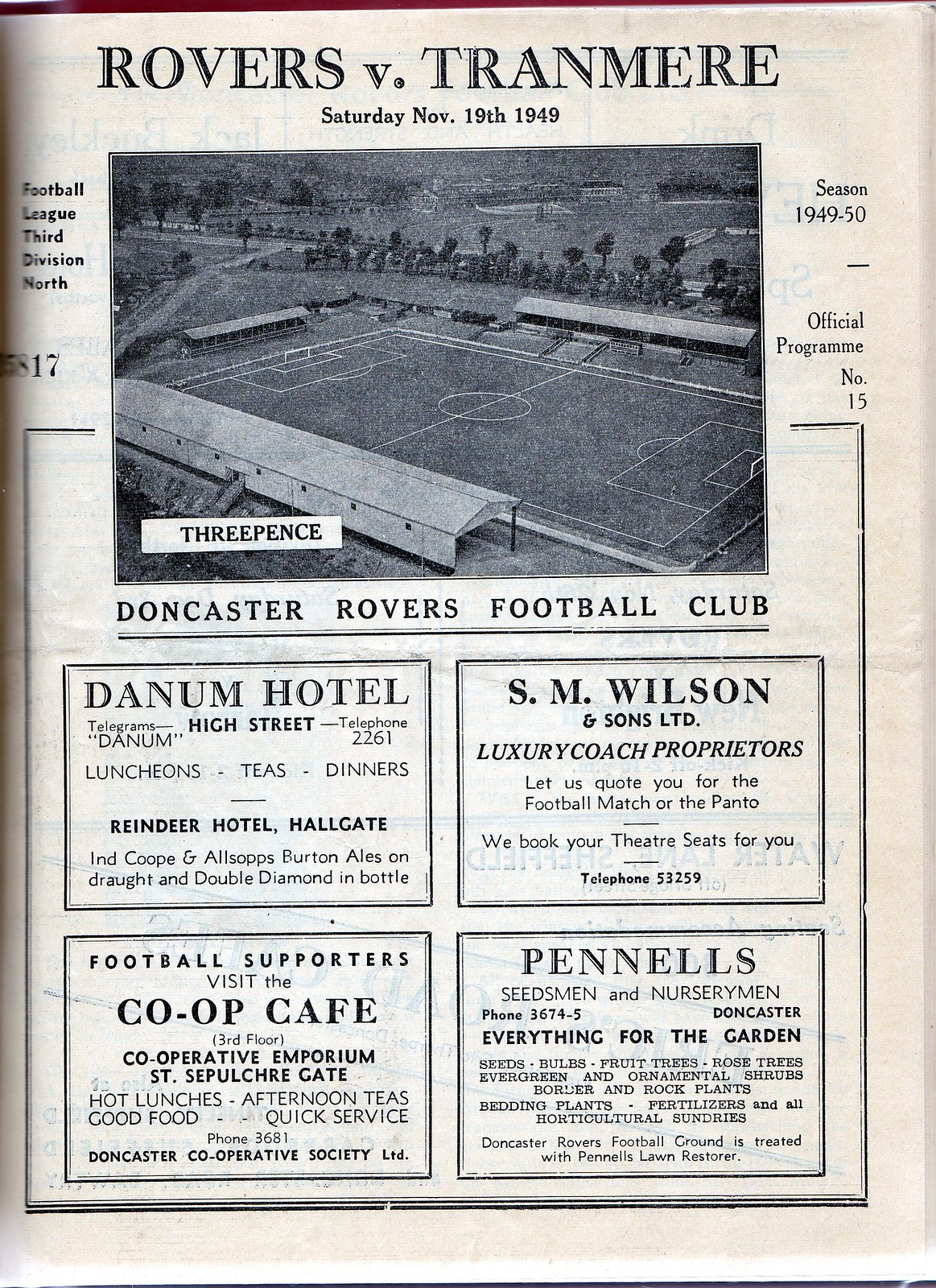This black-and-white image depicts the front page of an official match program for a soccer game between Doncaster Rovers Football Club and Tranmere Rovers, dated Saturday, November 19, 1949. This program, numbered 15 for the 1949-50 season, features the title "Rovers versus Tranmere" prominently at the top, with a picture of a soccer field. Above the field, it mentions Football League, 3rd Division North. Below the picture, it announces the Doncaster Rovers Football Club. The bottom half of the page is occupied by four business card-sized advertisements. These ads include the Danham Hotel on High Street, S.M. Wilson and Sons Limited, luxury coach proprietors, the Co-op Cafe which supports the football team, and Pennell’s Seed Men and Nursery Men, offering everything for the gardener. The layout of this nostalgic piece provides a glimpse into the graphic design and advertising styles of the late 1940s.